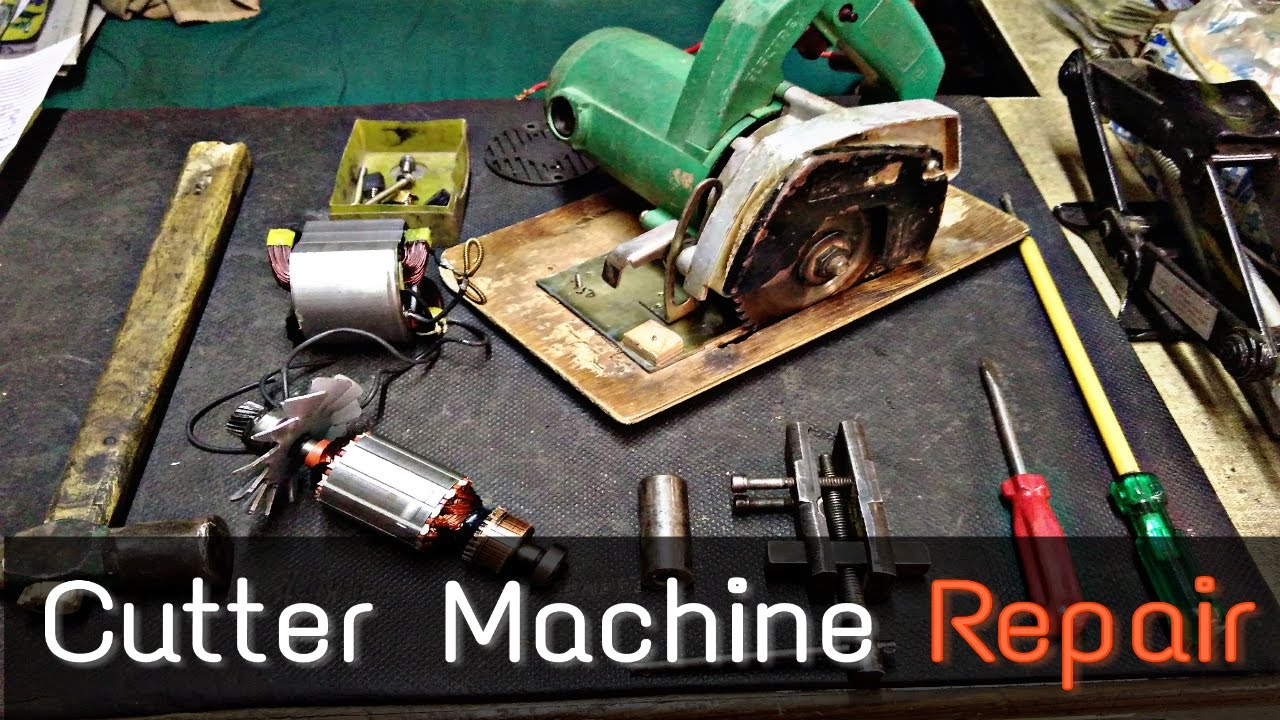This detailed photograph captures a meticulously organized workbench scene. Central to the image is a green planing machine, flanked by a second planing machine in black to the right. Surrounding these primary tools, a variety of other hardware is neatly laid out on a dark surface. Highlighted among these are red and green screwdrivers, metallic gray wrenches, a hammer, and a bit for a drill. Additionally, a circular saw is prominently placed above the text, which reads "Cutter machine repair"—with "cutter machine" in white and "repair" in orange. A yellow box containing several visible screws is situated further back, adding to the array of tools. In the background, a green fabric partially covers the table, suggesting an active and organized workshop environment specific to cutting and repairing machinery.